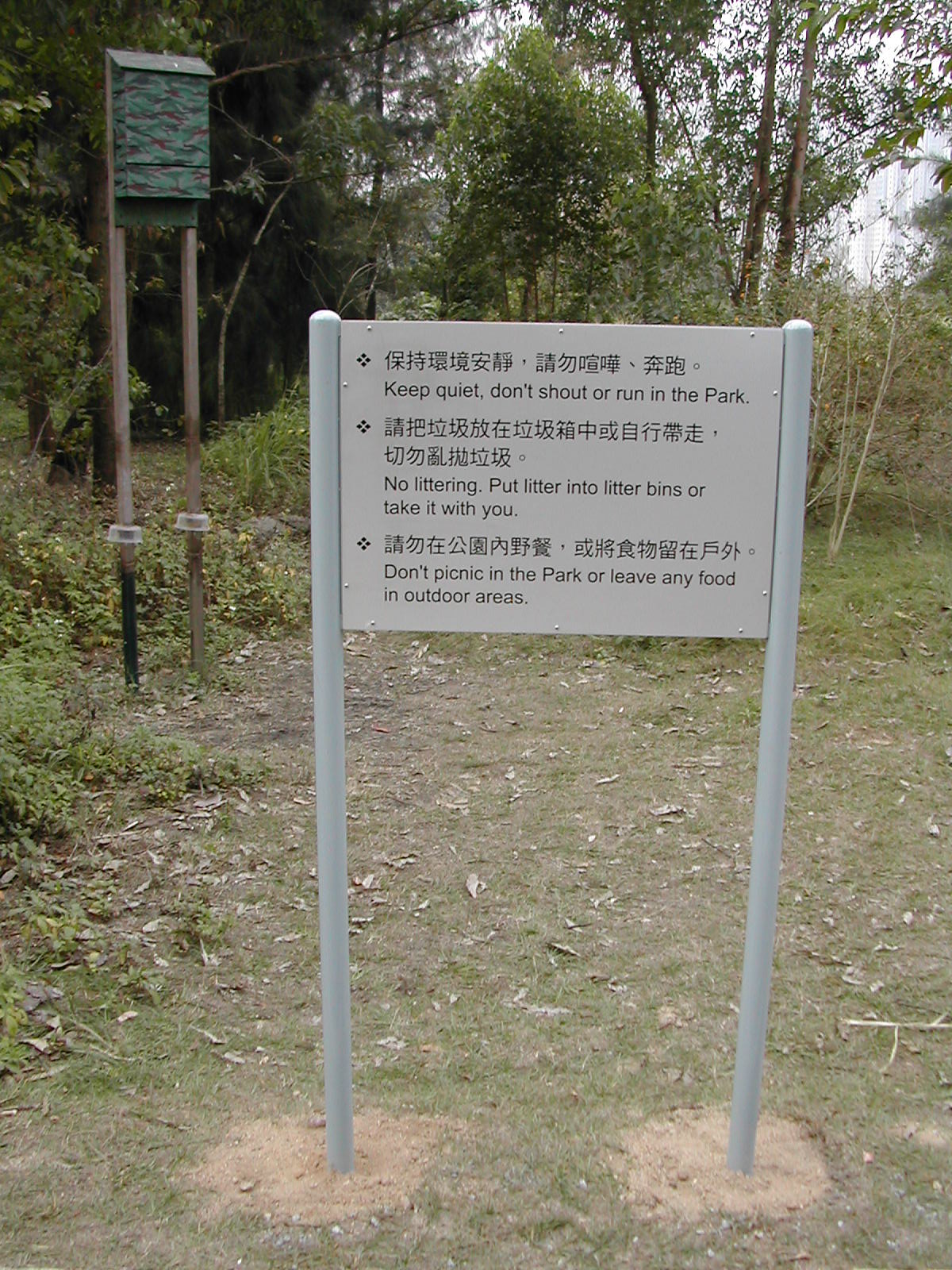This picture captures a white sign supported by two white poles, embedded in a grass-dirt ground. The ground appears flattened from frequent foot traffic, with patches of grass interspersed. To the left, in the upper part of the image, another sign is visible in the background. This secondary sign, mounted on brown posts, is predominantly green and might signify an entrance to a location, although its text is unclear due to the distance. Surrounding the area are trees, shrubs, and some small ground lights enhancing the natural ambiance.

The primary sign, written in Chinese symbols with English translations below, displays several cautionary guidelines for park visitors. The top line instructs, "Keep quiet, don't shout or run in the park." The second line advises, "No littering, put litter into litter bins or take it with you." The third line warns, "Don't picnic in the park or leave any food in outdoor areas." This sign appears to be situated at the entrance of an animal preserve, stressing important rules to ensure the safety and cleanliness of the park environment.